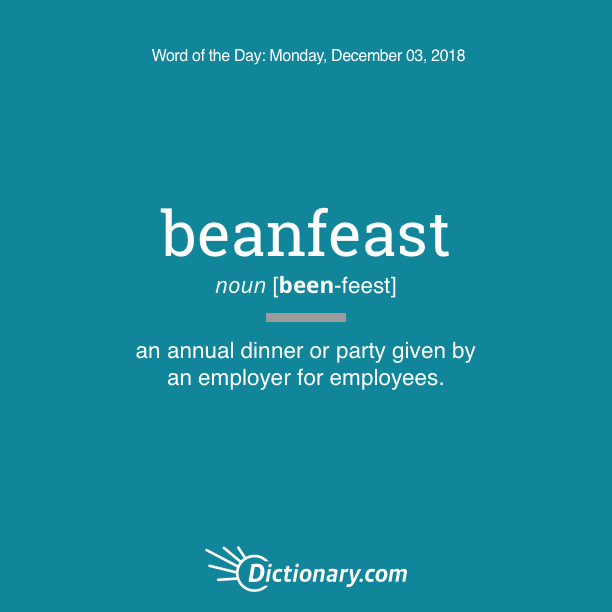The image is a perfectly square post, likely from Instagram, with a simple, matte light blue or teal background. At the very top, in small white letters, it reads "Word of the Day, Monday, December 3rd, 2018." Below this prominent header is the word "bean-feast" in larger white text. Directly underneath, in smaller white text, it specifies that "bean-feast" is a noun, and provides its pronunciation as "bin-feast." A small gray line separates this information from the definition below, which states, "an annual dinner or party given by an employer for employees." At the very bottom of the image is the dictionary.com logo, indicating the source of the Word of the Day.